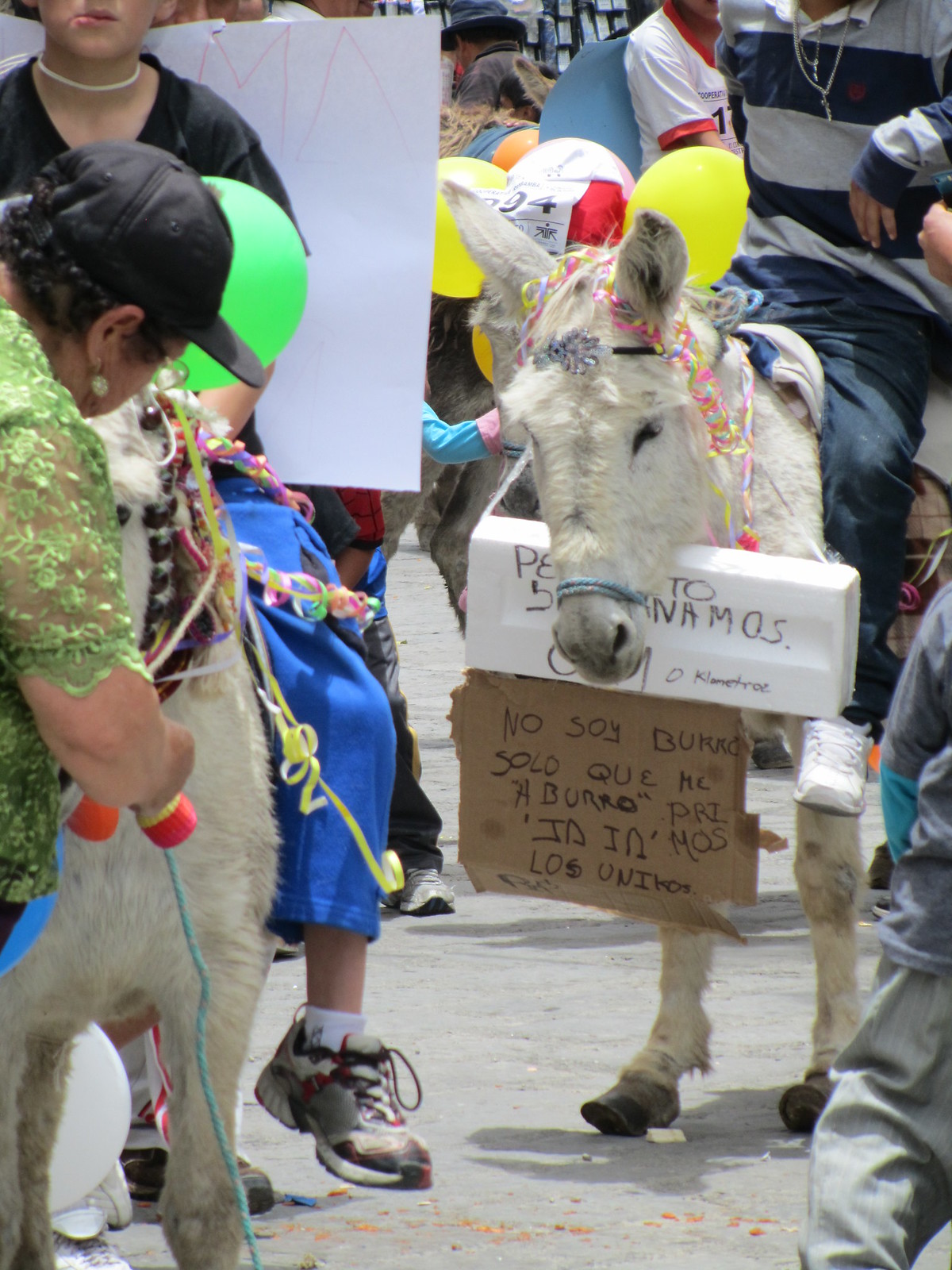In this vibrant photograph, two donkeys take center stage, surrounded by a group of people. The donkey on the right is striking with its white fur and black hooves, adorned with a styrofoam sign and a cardboard sign, both inscribed in Spanish using black marker. The signs hang prominently around its neck. This donkey also has colorful balloons attached above its head, as well as an official entrance number "94" visible on a white piece of paper above its right ear. A person, dressed in black pants and a grey and blue striped polo t-shirt, is seated on its back.

To the left, another donkey shares the scene, partially visible with a balloon tied above its head and its face slightly turned. This donkey is being attended to by a woman in a green top, who appears to be adjusting bright red adornments beneath its halter. The person riding this donkey wears a black shirt and blue pants around the animal's ears. Multiple multicolored ribbons add to the festive and lively atmosphere of the image.